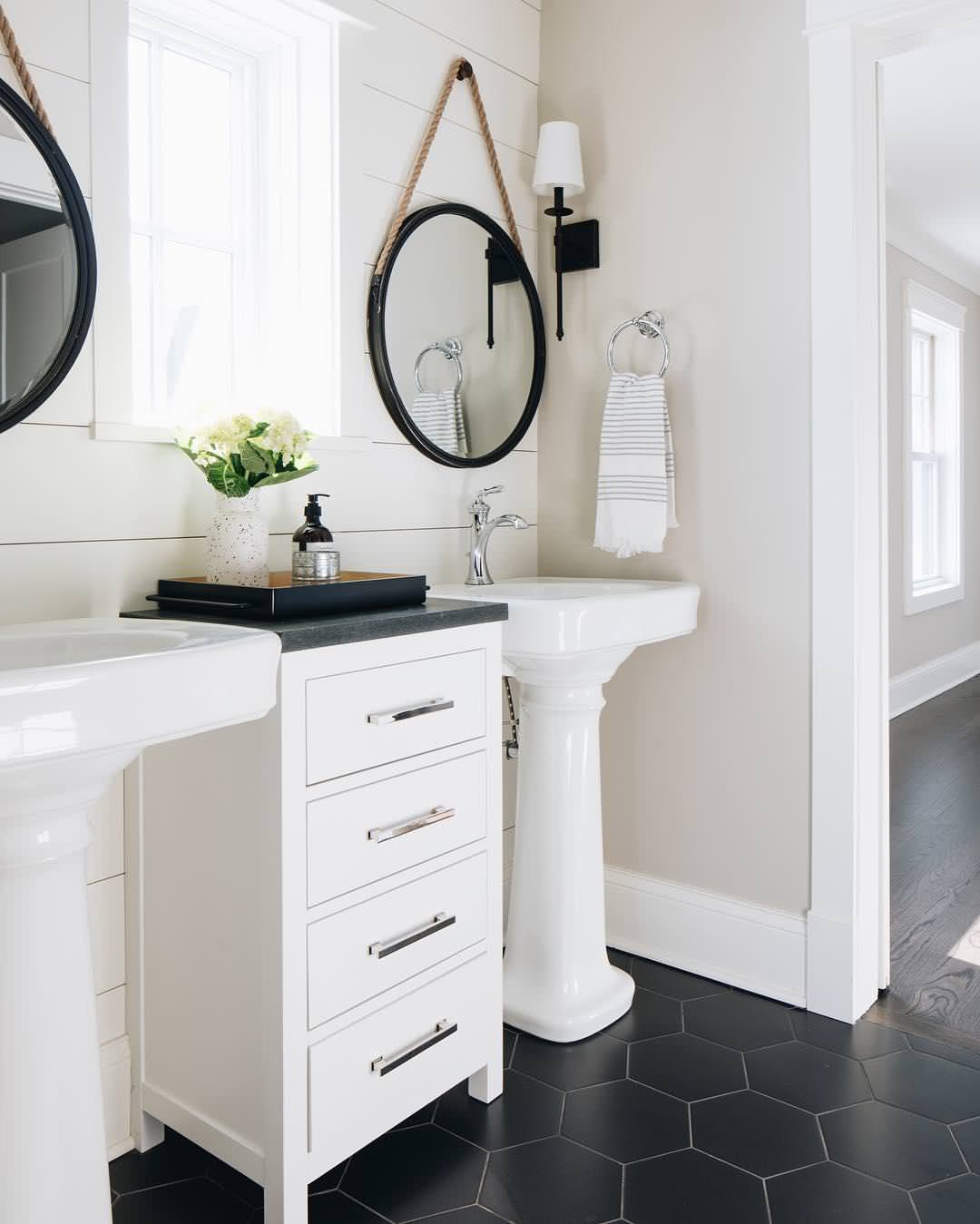The image showcases a pristine bathroom with a sophisticated design. The walls are adorned with white wooden shiplap panelling, complemented by medium to light white cream-based molding. Central to the scene are two standalone sinks flanking a white dresser-like counter space with four drawers, each accented by silver hardware pulls. The countertop is gray, topped with a stylish tray holding a soap dispenser and a vase of flowers. Above each sink hang round, black-framed mirrors suspended by ropes, adding a touch of rustic elegance. Between the sinks, set slightly to the left of the frame, is a window that allows natural light to brighten the space. A circular towel ring near one of the sinks holds a white striped dish towel, beneath a wall-mounted lantern-like sconce that provides additional illumination. The floor features black tiles with intricate geometric patterns, adding a contemporary touch to this refined, dual-sink bathroom.